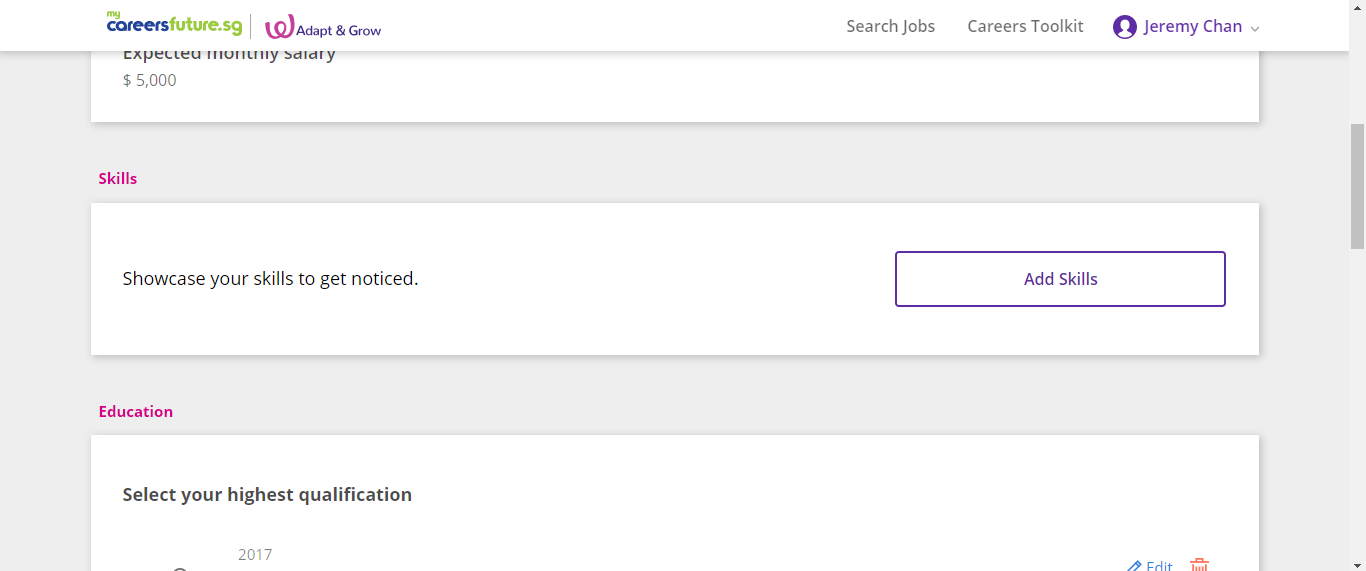The image has a white background with text elements and various colored sections and boxes. At the top, "Maya" is written in green, followed by "Careers" in blue, and "future.sg" again in green. A vertical gray line runs down the image, next to which there is a magenta "W." The phrase "Adapt & Grow" is written in purple. On the right-hand side, in gray text, it says "Search Jobs, Career, Toolkit." Below that, "Jeremy Chain" is written in purple.

The background then transitions to gray, overlaid with multiple white rectangular boxes. The first box is partially cut off at the top. Within most of these boxes, the text is in black. One prominent detail is "Expected Monthly Salary," which is indicated as $5,000. Below this, in the gray space, "Skills" is written in magenta on the left-hand side. Another white box states in black, "Showcase Your Skills to Get Noticed."

On the right-hand side of another box, which has a white interior and a purple border, the text reads in purple, "Add A Skills" with both 'A' and 'S' capitalized. There is some space between these elements. Further down, "Education" is written in magenta. Another box that is partially visible due to the image cut-off contains the text "Select Your Highest Qualification" on the left-hand side in black, with a notation of "Grade 2017" beneath it. On the right side, in blue, it appears to say "Edit," and near this is an icon resembling an orange and white trash can, presumably to delete an entry.